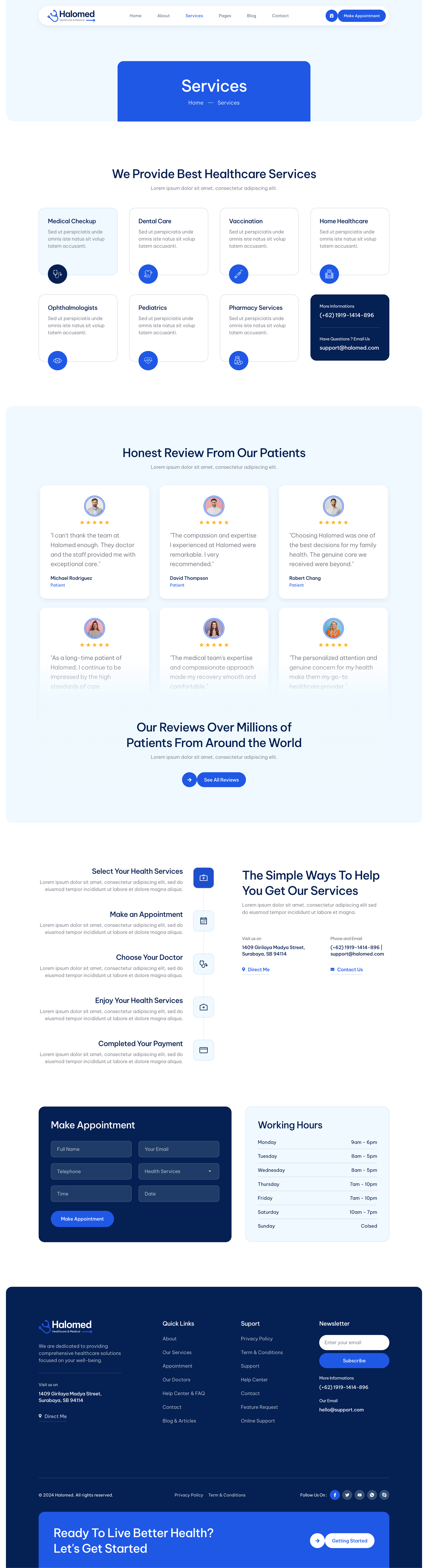This image depicts the website HaloMet, featuring a predominantly blue and white color scheme that incorporates various shades of these colors for visual interest. At the very top, there's a light blue header banner with a thin white tab above it. The white tab includes the HaloMet logo on the left and a navigation menu with the options Home, About, Services, Pages, Blog, and Contact. The "Services" tab is highlighted in blue, indicating that the current page being viewed is the Services page. To the right of the navigation menu, there's a darker blue button labeled "Make Appointment".

Beneath the header, there's a large blue box displaying navigation links for "Home" and "Services" against a white background. Below this, a white section prominently states, "We provide the best healthcare services." This area includes small boxes listing various services offered: Medical Checkup, Dental Care, Vaccination, Home Healthcare, Ophthalmology, Pediatrics, and Pharmacy Services. A box at the end provides a contact phone number and email for more information.

Further down, there's a blue box featuring testimonials titled "Honest reviews from our patients," with six white boxes that include a small photo of each reviewer, their rating, a comment, and their name. A statement underneath notes, "Reviews from millions of patients around the world," accompanied by a blue button to view all reviews.

Below this section is another white panel on the left, depicting a step-by-step guide titled "Select your health services." The steps listed are: Select your health services, Make an appointment, Choose your doctor, Enjoy your healthcare services, and Complete your payment. To the right, it reads, "The simple ways to help you get our service," with the address, phone number, and email provided.

Finally, at the bottom of the image, there is a blue box labeled "Make Appointment," alongside the website's working hours.